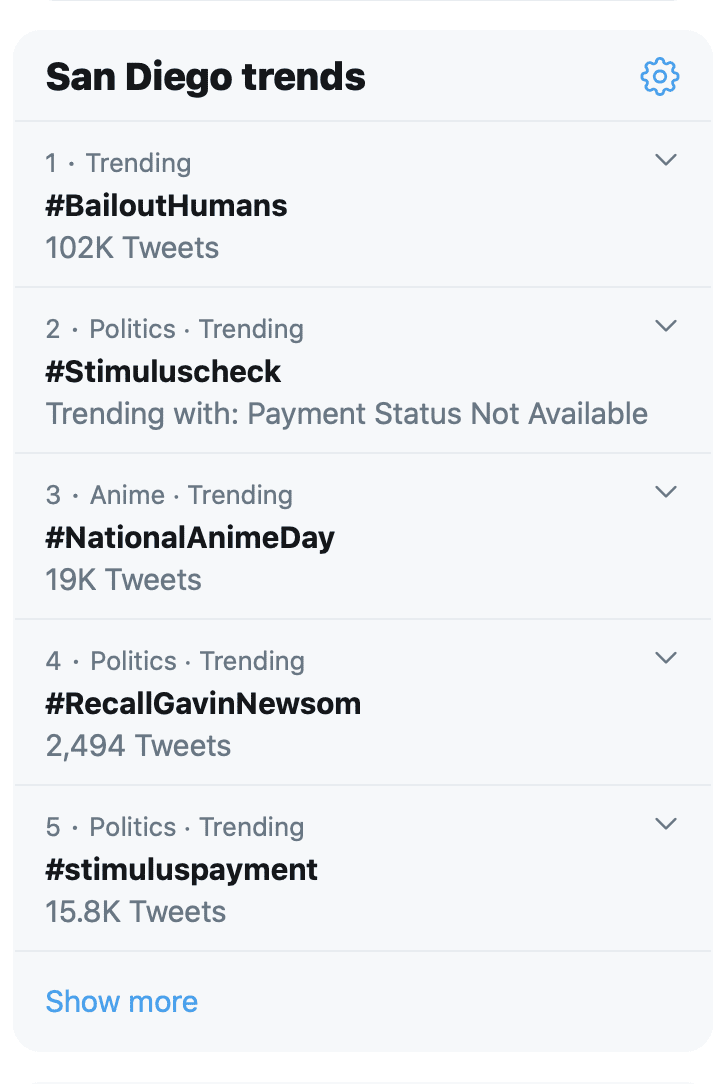This screenshot of the Twitter trending tab features a light blue background. At the top left, bold black text reads "San Diego Trends," while the top right corner displays a cogwheel icon for settings. The number one trending hashtag, "#BailoutHumans," boasts an impressive 102,000 tweets. Directly beside it to the right, a drop-down menu is visible. The second trend is categorized under "Politics Trending" and highlights the hashtag "#DemiLiszczyk." This entry is noted to be trending alongside "Payment Status Not Available," and also features an adjacent drop-down menu. In total, five trends are displayed in the screenshot, each accompanied by a drop-down menu on their right. At the bottom left of the screen, a blue-font link invites users to "Show more."